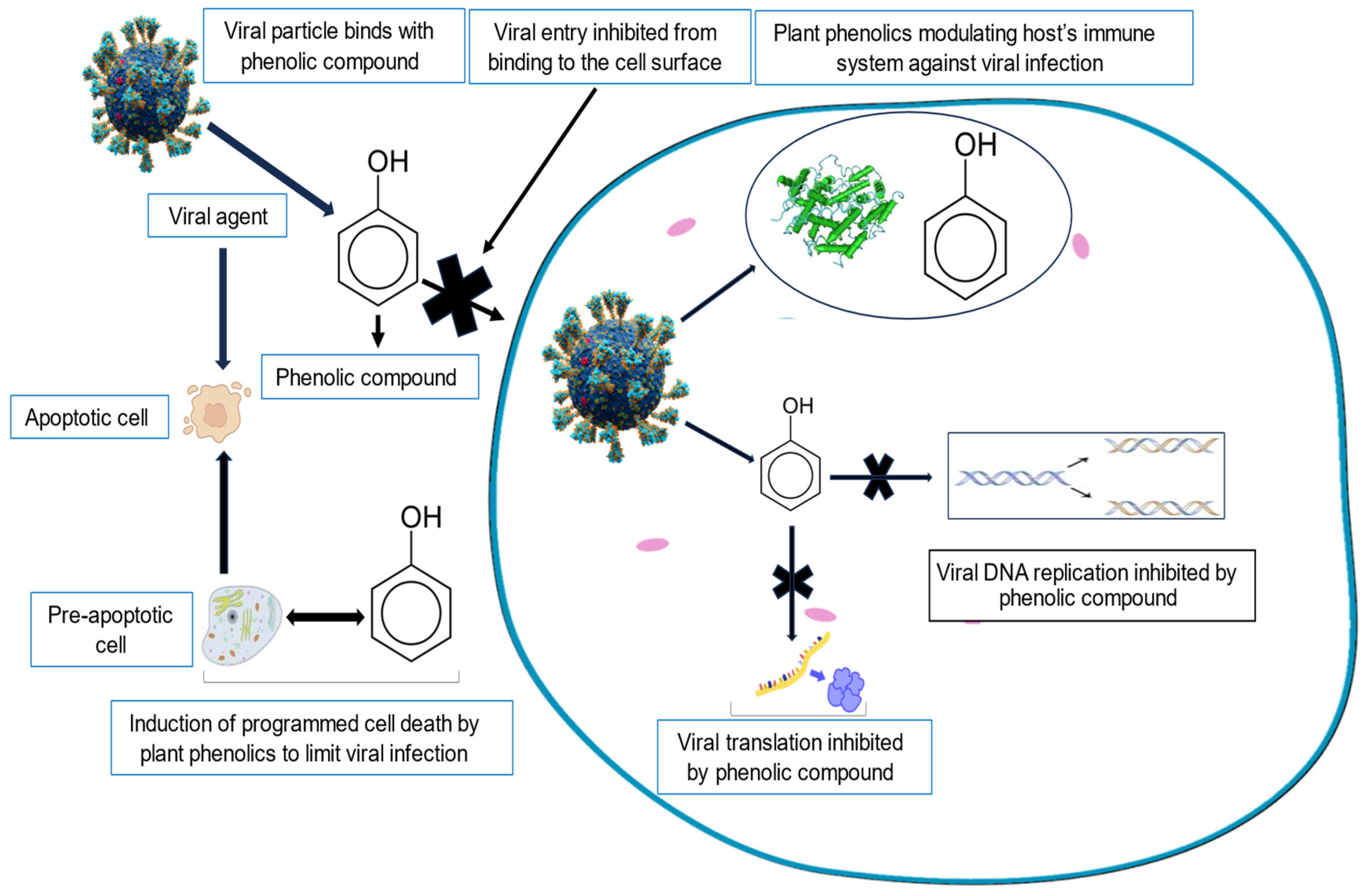The image resembles a science textbook illustration explaining the interactions between viral particles and phenolic compounds. On the left, there's a detailed 3D depiction of a blue viral particle with projections sticking out. It includes a downward diagonal pointer indicating a chemical structure labeled OH, representing an oxygen-hydrogen bond. Above this structure, there's text about a "viral agent" pointing towards a pink blob representing an apoptotic cell. To the right, a sequence of blue-bordered text boxes elaborates on the process: the first box mentions the "viral particle binds with phenolic compound," the next indicates "viral entry inhibitor from binding to the cell surface," and the third discusses "plant phenolics modulating the host immune system against viral infections." Further details include references to viral DNA replication and the inhibition of viral translation by phenolic compounds. Overall, it outlines how plant phenolics can prevent viral infection by modulating immune responses and inhibiting viral replication, with various scientific elements and pathways illustrated throughout the image.